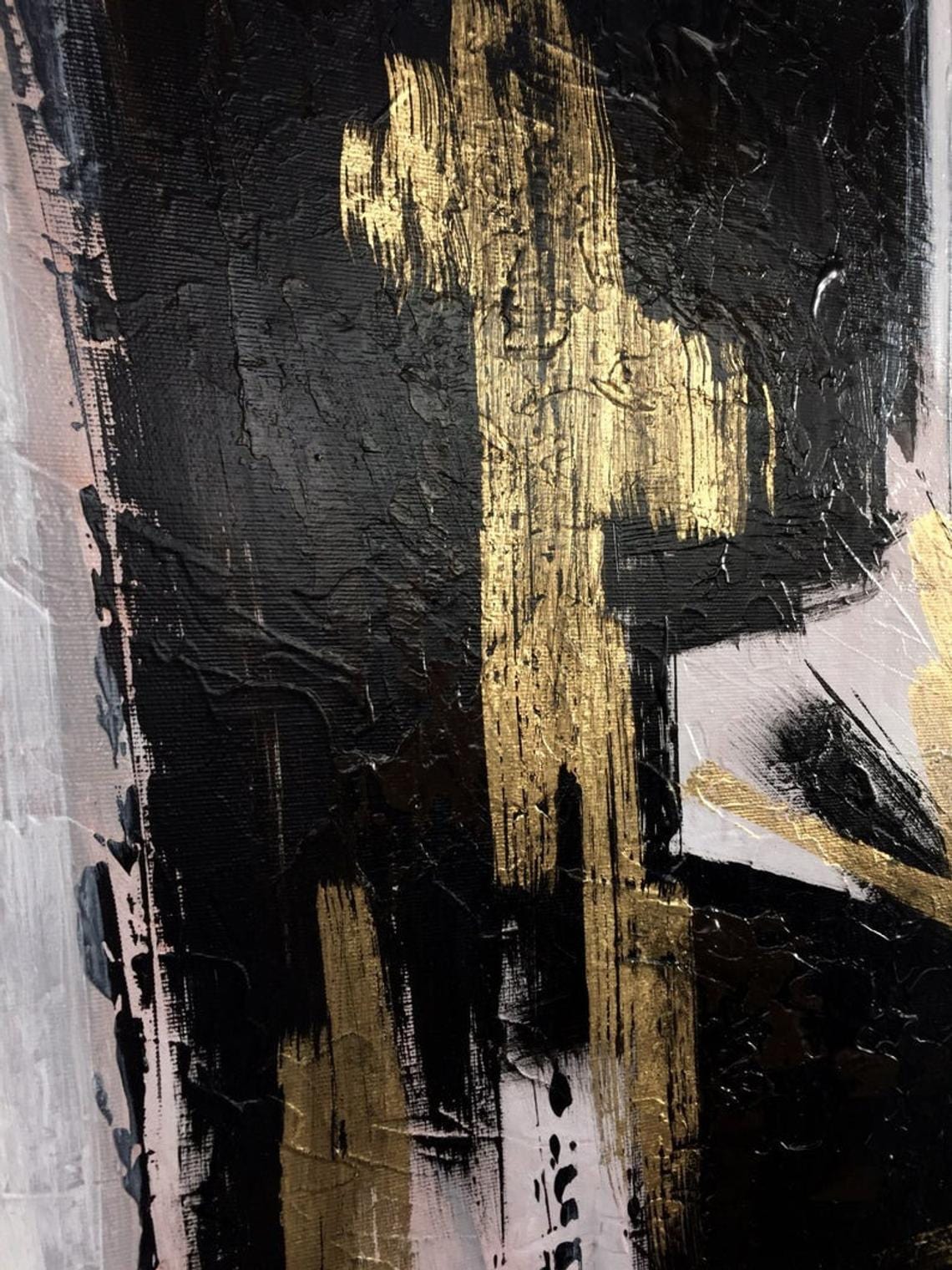This is a detailed close-up image of an abstract vertical oil painting, predominantly featuring black, white, and metallic gold colors, with additional hues of gray and pinkish tones. The black paint forms the primary background with heavy, shiny brush strokes, appearing textured as if they were applied over a crumpled surface. The topmost and central area showcases a prominent cross-like shape in gold paint. White and gold streaks are interspersed, especially noticeable on the far right and bottom foreground. The overall style is reminiscent of mid-20th century traditional abstract art, focusing on the texture and heavy brush strokes rather than depicting any decipherable shapes or forms.